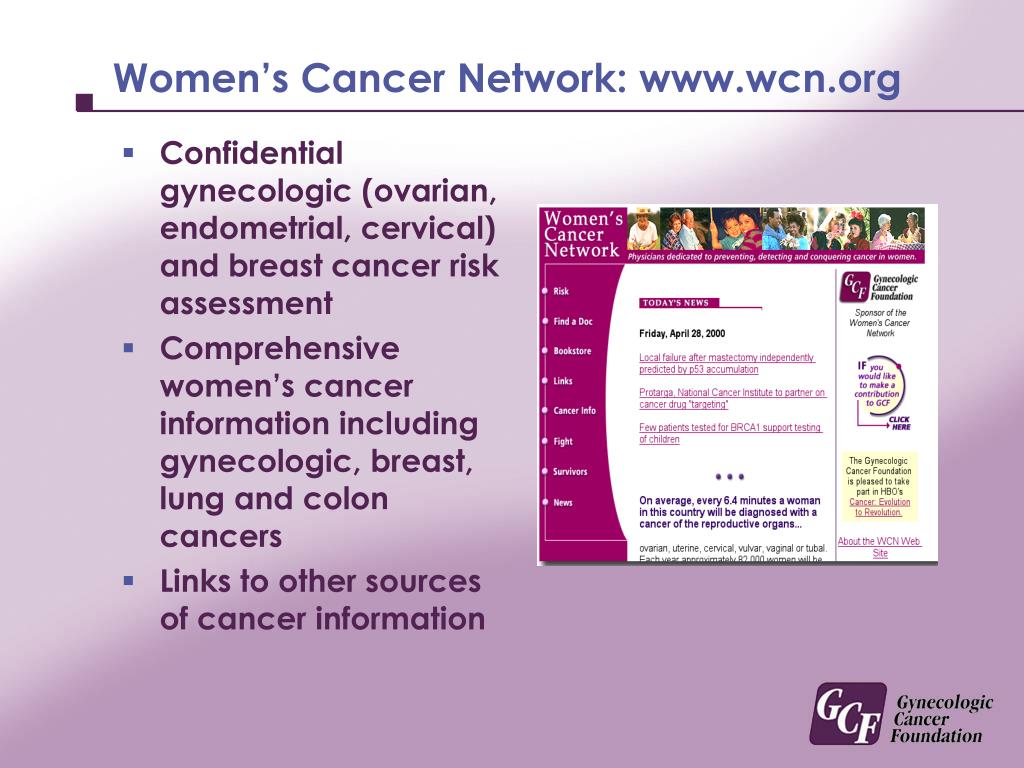This is a detailed screenshot of the Women's Cancer Network website. The background features a gradient transitioning from pinkish-gray at the top. In purple font at the top of the page, it reads: "Women's Cancer Network: www.wcn.org." Below this header is a black line that demarcates the start of the content.

Under the black line, there is a bullet list. The bullets are purple squares, followed by text in black font. The first bullet point states: "Confidential Gynecologic, Ovarian, Endometrial, Cervical, and Breast Cancer Risk Assessment." The second bullet reads: "Comprehensive Women's Cancer Information including Gynecologic, Breast, Lung, and Colon Cancers." The third bullet says: "Links to Other Sources of Cancer Information."

To the right of the bullet list, there is a small screenshot of another part of the website being advertised. At the top of this inset image, it again says "Women's Cancer Network" along with several small photographs of women affected by cancer. Below this, in block text, it reads: "Physicians Dedicated to Preventing, Containing Cancer in Women." 

On the left side of the inset image, there is a vertical menu listing various options: "Risk," "Find a Doc," "Bookstore," "Links," "Cancer Info," "Fight," "Survivors," and "News."